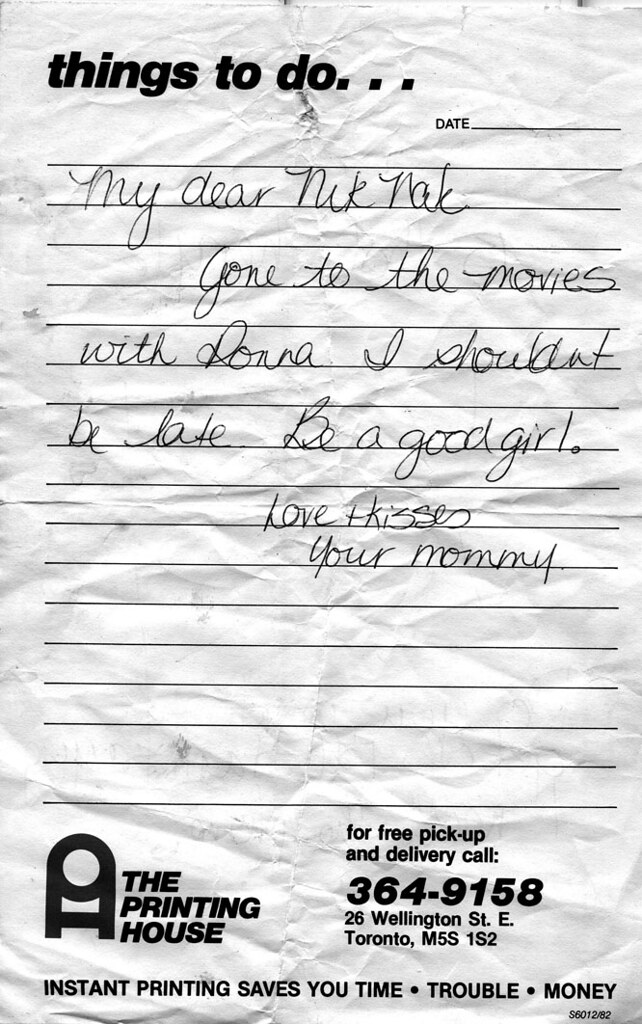The image depicts a black-and-white scan of a crumpled, torn-out notepad page, likely folded and rolled at some point. The top of the ruled paper reads in bold font, "Things to do...". To the upper right, there's the word "Date" with a blank line beside it. The page features approximately 20 evenly spaced horizontal lines running across it. Written in cursive pen, the note reads: "My dear Nick-Knack, gone to the movies with Donna. I shouldn't be late. Be a good girl. Love and kisses, your mommy." The bottom left corner showcases a logo and the name "The Printing House." Adjacent to it, on the bottom right, the text reads: "For a free pickup and delivery call 364-9158, 26 Wellington Street East, Toronto M5S 1S2. Instant printing saves you time, trouble, money." This detailed note appears to be a mother's message to her daughter, Nick-Knack, explaining her absence and urging good behavior.